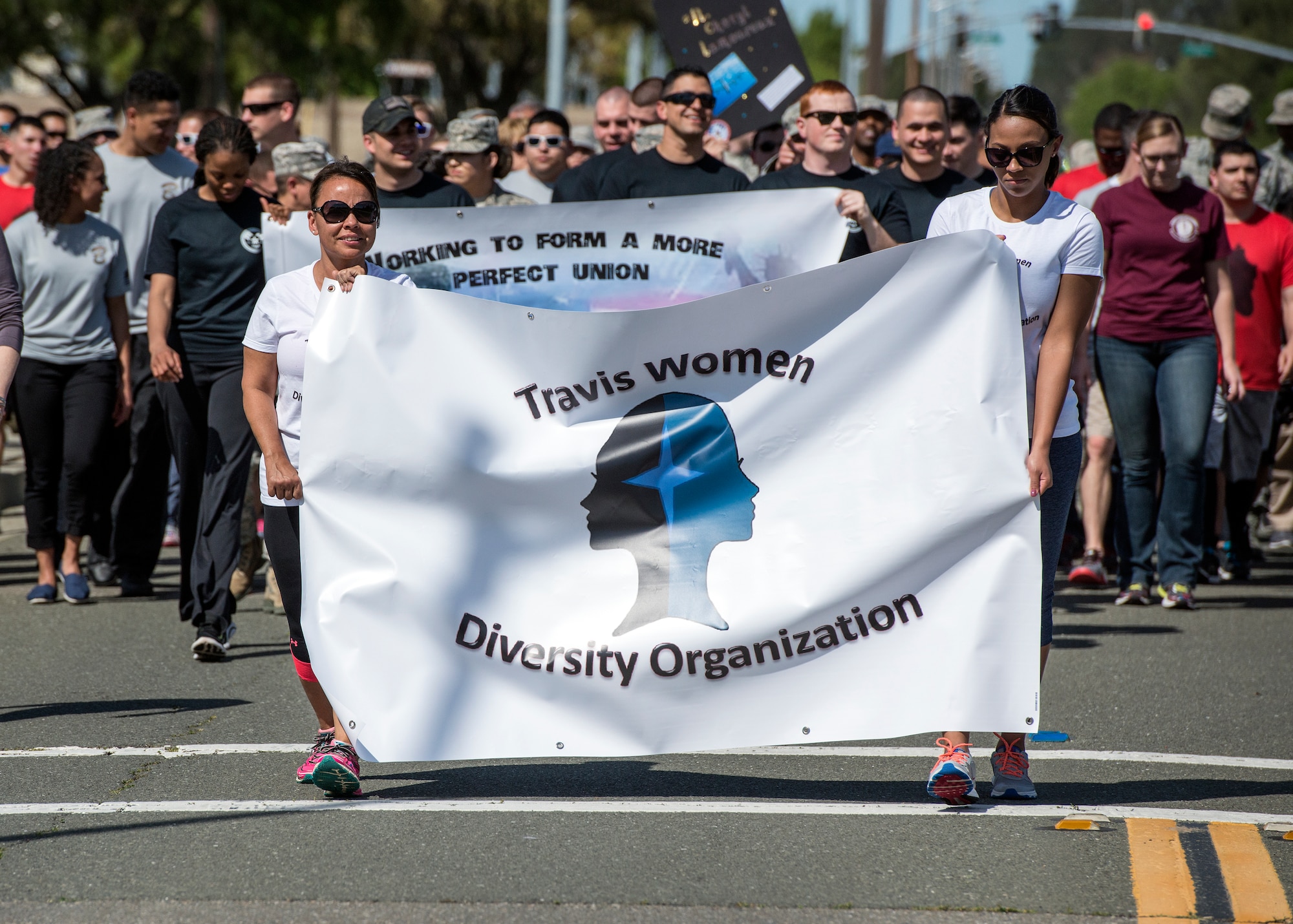This photograph captures a vibrant parade organized by the Travis Women Diversity Organization, set against a bustling city street during the daytime. At the center of the image, two women of color, both with light brown skin and black hair, stand prominently behind a large white banner that reads "Travis Women Diversity Organization" in black text. The banner also features a logo with two women's silhouettes—one black facing left and one blue facing right—separated by a four-pointed star. The women, dressed in white short-sleeved t-shirts, dark yoga pants, running shoes, and big dark sunglasses, are positioned in a white crosswalk that intersect a road marked with a double yellow line.

In the background, a diverse crowd of men and women can be seen marching, including individuals holding another banner that states, "Working to Form a More Perfect Union," accompanied by an American flag. Among the crowd are several soldiers in camouflage uniforms. The scene is framed with the city’s infrastructure, including traffic lights and street signs in the distance, and is flanked by trees lining the sides of the street. The photo encapsulates the spirit of unity and diversity as the participants march together.